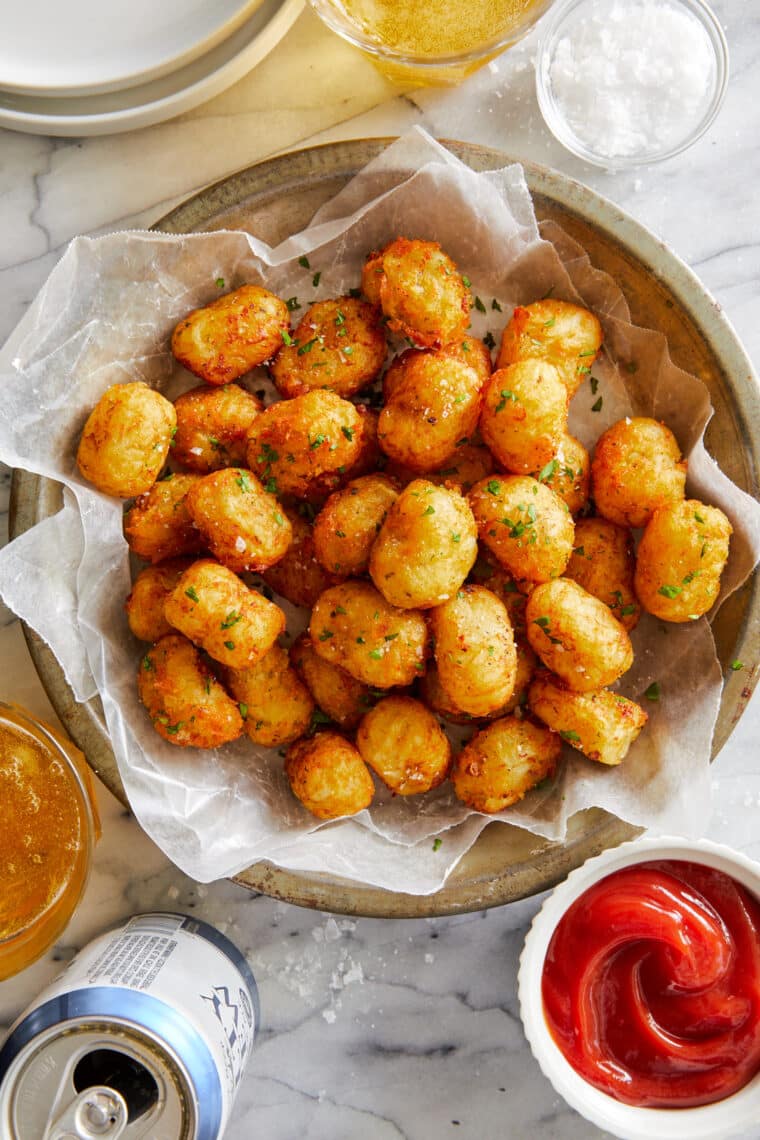This close-up photograph captures a richly detailed scene on a white and black marbled countertop. Central to the image is a light brown clay bowl lined with parchment paper, showcasing a generous serving of golden brown, crispy, breaded snacks that resemble tater tots. These snacks are garnished with an unidentified green seasoning. To the immediate right of the bowl, a white ceramic dish holds a deep red ketchup elegantly swirled like a wave. Additionally, a small glass dish filled with salt sits in the top right corner. On the bottom left, a cyan blue and white beer can with an open top and a hint of condensation on the rim is visible, alongside a glass partially filled with an orange liquid. Tucked in between, there is another glass dish containing a yellow liquid, rounding out the tantalizing array of accompaniments.